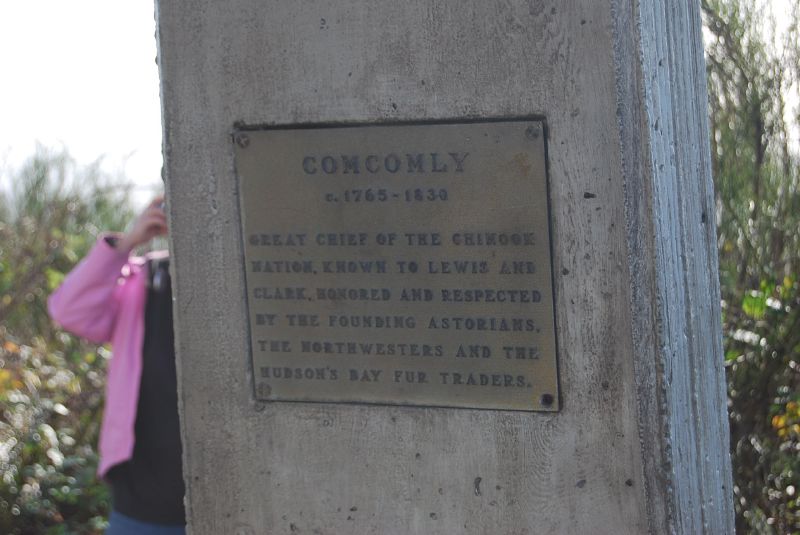The photograph captures an outdoor scene, featuring a large, vertically-oriented wooden pillar, partially framed against an overcast sky. Affixed to the pillar is a rectangular metal plaque with a silvery bronze hue, secured by four bolts at each corner. The plaque bears the inscription: "Comcomly, 1765 to 1830. Great Chief of the Chinook Nation known to Lewis and Clark, honored and respected by the founding Astorians, the Northwesterners, and the Hudson Bay fur traders." Surrounding the wooden structure are tall green shrubs and branches. In the background, on the left side of the image, a person is partially visible, wearing a pink jacket and a black shirt, seemingly engaged in a phone conversation.